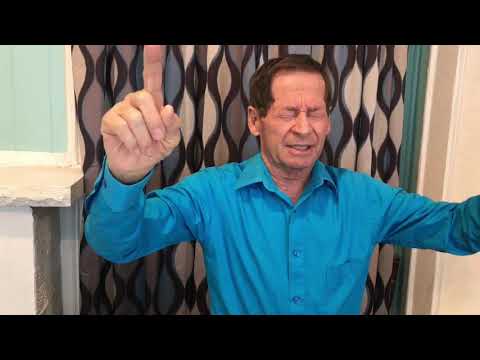A man is prominently featured in this image, which has a thick black border at the top and bottom. He appears to be either sitting or standing in a relaxed setting, possibly during an online sermon or similar activity. He has closed eyes, short brown hair, and is wearing a long-sleeved, button-up turquoise blue shirt. His head is tilted slightly to the right, and his mouth is partially open as if mid-speech. Both of his arms are raised to shoulder level; his left arm extends out of the frame while his right arm, with the index finger pointing upwards, creates a semi fist.

The background consists of a cool, brightly lit room with light-colored walls. A ledge is visible on the left side of the image. Behind the man, there are distinctive draperies featuring brown, white, blue, purple, and pink vertical patterns. This decorative curtain lies between two wall sections, adding a touch of complexity and color to the scene. Despite the slight ambiguity around his exact posture, the setting exudes a sense of comfort and tranquility.